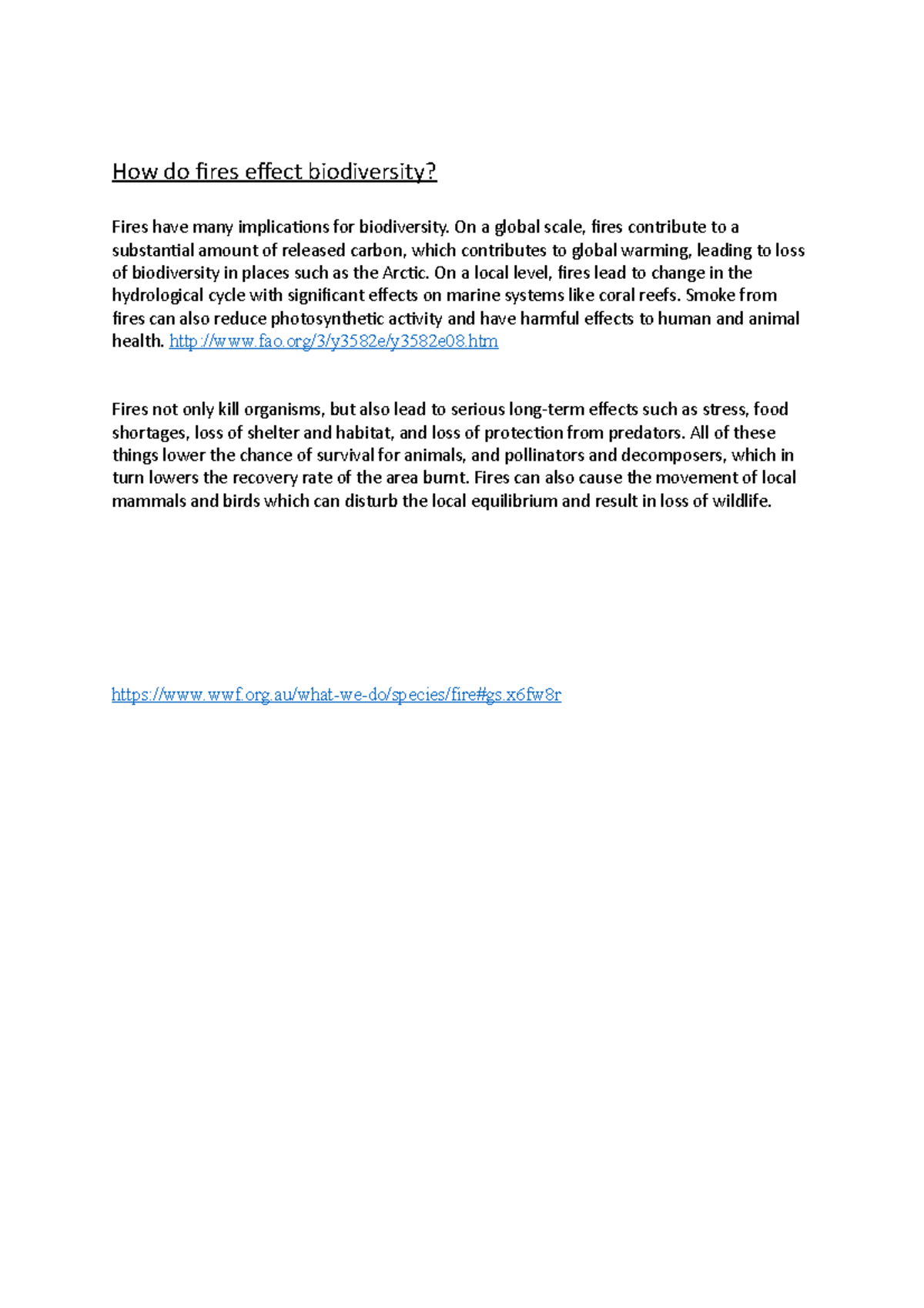The image features a clean, all-white background. In the top left corner, larger black lettering poses the question, "How do fires affect biodiversity?" with a black line underneath it for emphasis. 

Beneath this heading is a detailed paragraph spanning six lines in black text. It reads: "Fires have many implications for biodiversity. On a global scale, fires contribute to a substantial amount of released carbon, which contributes to global warming, leading to loss of biodiversity in places such as the Arctic. On a local level, fires lead to changes in the hydrological cycle with significant effects on marine systems like coral reefs. Smoke from fires can also reduce photosynthetic activity and have harmful effects on human and animal health."

Below this paragraph, a clickable blue link offers more information. 

After a small space, another five-line paragraph in black text follows: "Fires not only kill organisms, but also lead to serious long-term effects such as stress, food shortages, loss of shelter and habitat, and loss of protection from predators. All of these factors lower the chances of survival for animals, pollinators, and decomposers, which in turn lowers the recovery rate of the burnt area. Fires can also cause the movement of local mammals and birds, disturbing the local equilibrium and resulting in the loss of wildlife."

Finally, at the bottom left corner of the image, a second clickable blue link is provided for additional information.